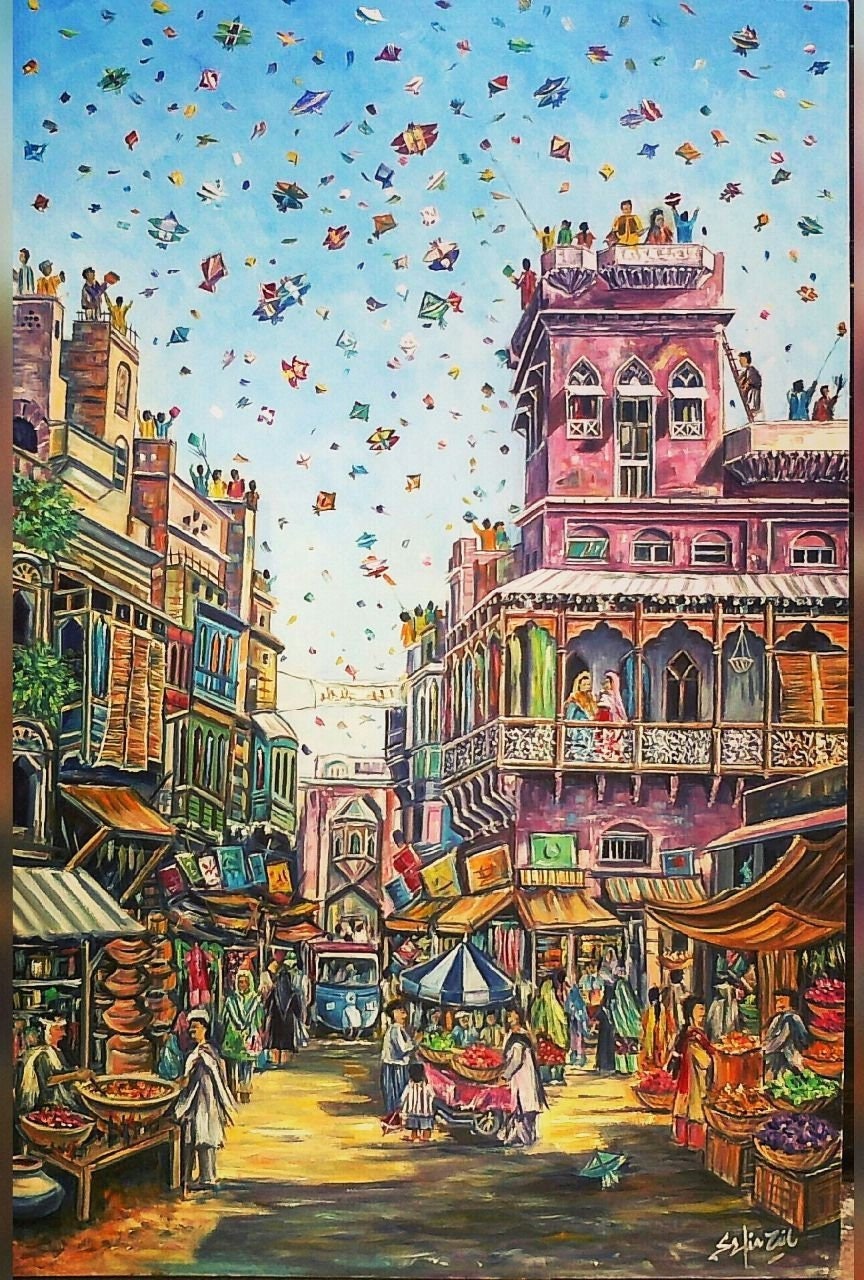This vibrant painting depicts a bustling and festive city scene, likely of Mediterranean or European inspiration, filled with the rich colors of pink, green, and blue. The scene unfolds in a busy district bustling with activity, featuring two- and three-story buildings adorned with lively hues of pink, brown, and blue. The streets are teeming with people, many dressed in white with white hats, alongside others in yellow and orange outfits, engaging in lively market exchanges. Tables are set up outside, showcasing a variety of goods, from produce reminiscent of a farmer's market to baskets and other market wares. Above, the sky is ablaze with colorful streamers and confetti-like items in red, blue, and green, enhancing the celebratory atmosphere. Some spectators can be seen on the second-floor balconies, watching the vibrant street scene below. An umbrella with a blue and white tent top adds to the festive aesthetic. The scene encapsulates the joyous essence of a city's market day, suggesting a fun, lively occasion where visitors and locals alike have gathered to celebrate.